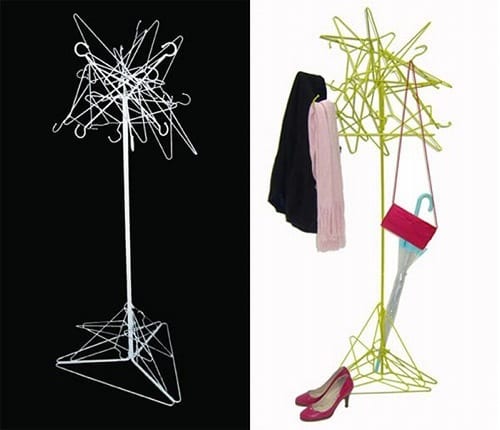The image features a split-screen design, showcasing two versions of the same coat hanger stand. On the left side, against a black background, stands a white coat hanger rack, resembling a tree made entirely of tangled white coat hangers. The stand is chaotic, with hangers haphazardly entwined, creating a striking contrast with the dark backdrop. The right side reveals the same scene but in vibrant color. Here, the background is white, illuminating a lime green coat hanger stand adorned with various items. Draped over the scattered hangers are a pink scarf and a black scarf. A red purse hangs prominently, while a blue and white umbrella leans against the base of the stand. At the foot of the rack lies a pair of red high heels, adding a final touch of vivid color to the composition.